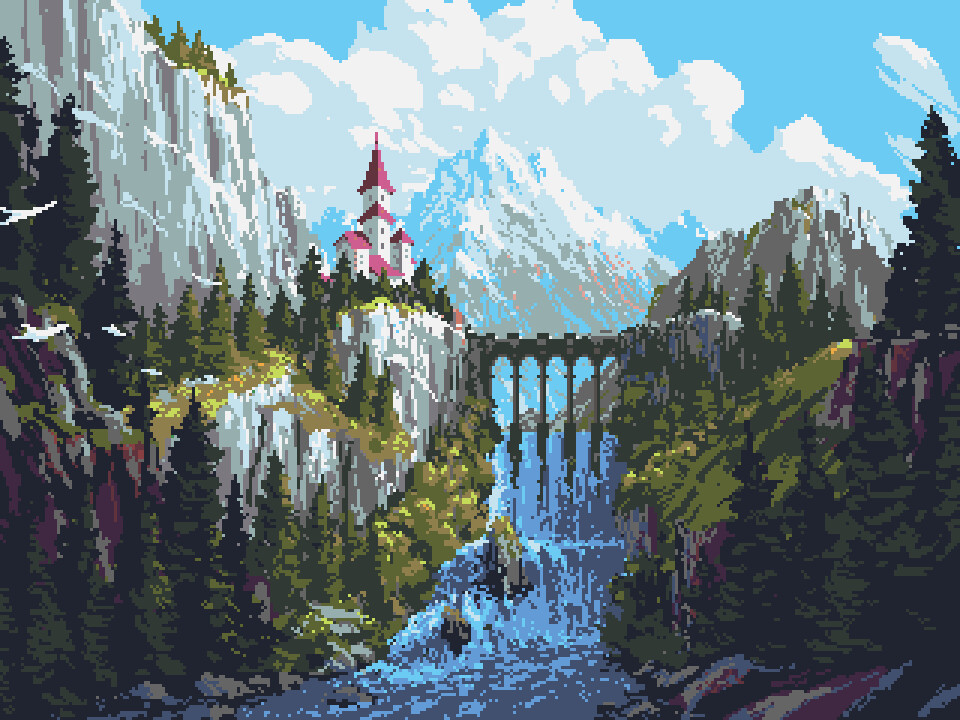The image depicts a pixel art landscape featuring a centrally positioned waterfall with a bridge arching across it. Above the waterfall, a bridge spans from one side of the expanse to the other. To the left of the waterfall, in the distance, there is a pink and white castle with a red spire. Surrounding this castle are pine trees and mountainous terrain. The mountains to the left and right of the waterfall are detailed with snow-capped peaks in white and gray hues, adding to the scenic backdrop. Toward the top of the image, especially in the center and extending to the upper right, a blue sky dotted with white clouds is visible. Additionally, there appear to be some white birds flying around the middle left section of the image. The overall view is pixelated, giving it an artistic, computer-generated quality.